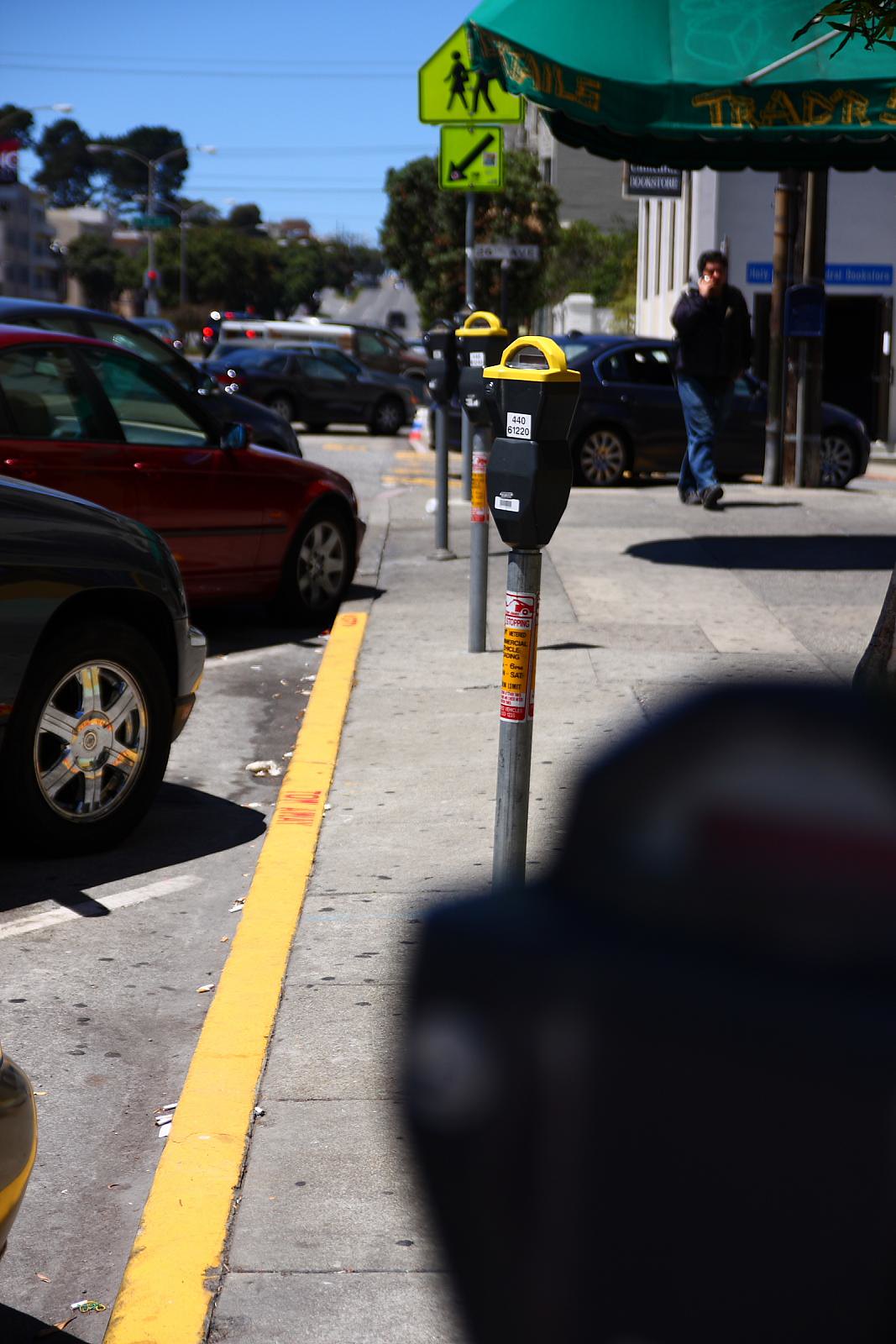This is a detailed photograph of a town street, focusing on a series of parking meters along a concrete sidewalk. The image, taken from a low angle at the edge of the sidewalk, prominently features a blurred black parking meter in the immediate foreground. This meter, out of focus due to its proximity to the camera, is mounted on a silver pole. Slightly behind, two more parking meters stand clearly visible on silver poles with orange stickers. These meters are black with yellow and white detailing on the top. Parked cars can be seen on the left, lined up in front of the meters along the yellow-painted curb, adorned with red letters.

A male pedestrian with pale skin and dark, short hair is walking on the sidewalk in the background. He is wearing blue jeans and a black jacket, holding a cell phone to his ear. Further up the sidewalk, a dark green awning with gold lettering and a crosswalk warning sign featuring a yellow background with a black silhouette of a parent and child can be seen. Below this sign is another, a black square with a black arrow pointing diagonally downward to the left. The concrete sidewalk is dotted with black spots, likely old gum or debris. The overall scene captures a typical urban setting with a mixture of pedestrian activity and parked vehicles.